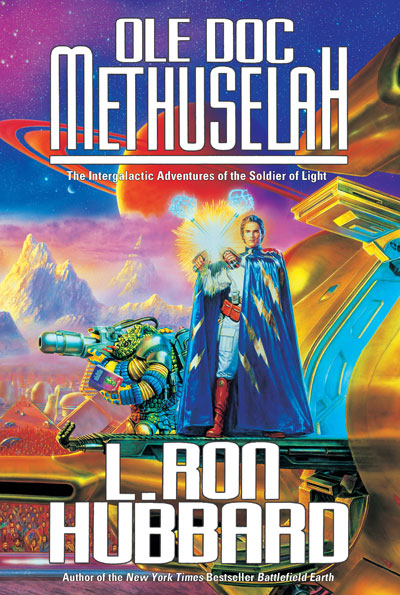The image is a vibrant and detailed book cover by L. Ron Hubbard, prominently featuring his name at the bottom in bold white, all-caps letters, accompanied by the subtitle "Author of the New York Times Bestseller, Battlefield Earth." The top of the cover showcases the book's title, "Old Doc Methuselah," written in all caps with an underline, followed by the tagline, "The Intergalactic Adventures of the Soldier of Light." The central artwork displays a heroic figure adorned in a striking blue cape embellished with gold lightning bolts, a blue shirt, and red belt, boots, and pants. He stands on a platform reminiscent of the portals seen in the movie Thor, with his fists raised and emanating clouds of smoke. The background features the ringed planet Saturn and other celestial bodies, amidst a starlit sky and distant white-gray mountain peaks. Next to him is a curious character that combines features of a lizard and a rhino, engrossed in reading a book. Additionally, a robotic creature crawls in the foreground, adding to the cover’s fantasy and sci-fi elements, while another figure peers through a telescope, enhancing the sense of adventure and exploration.